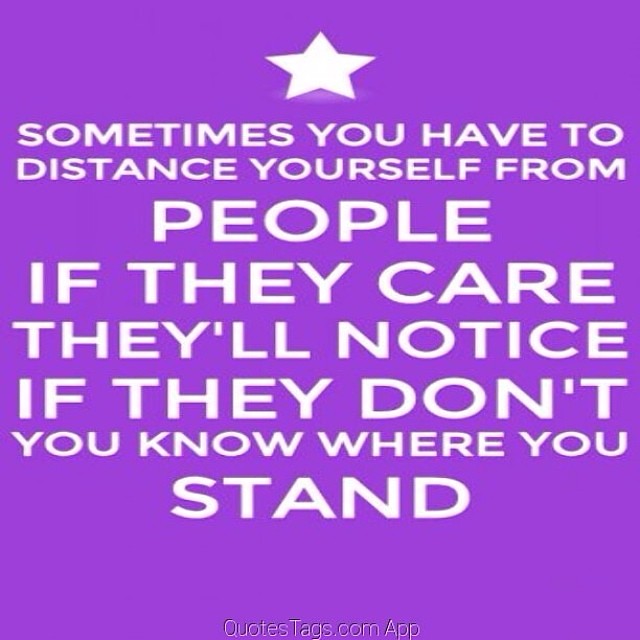The image is a square poster with a bright purple background. At the top center, there is a prominent white star. Below the star, the main quote is written in white font with varying sizes of text. The quote reads, "Sometimes you have to distance yourself from people. If they care, they'll notice. If they don't, you know where you stand." At the very bottom of the poster, in small white text, it reads "QuotesTag.com App." The lack of punctuation throughout the quote makes it challenging to interpret, emphasizing the need to read it carefully for clarity.